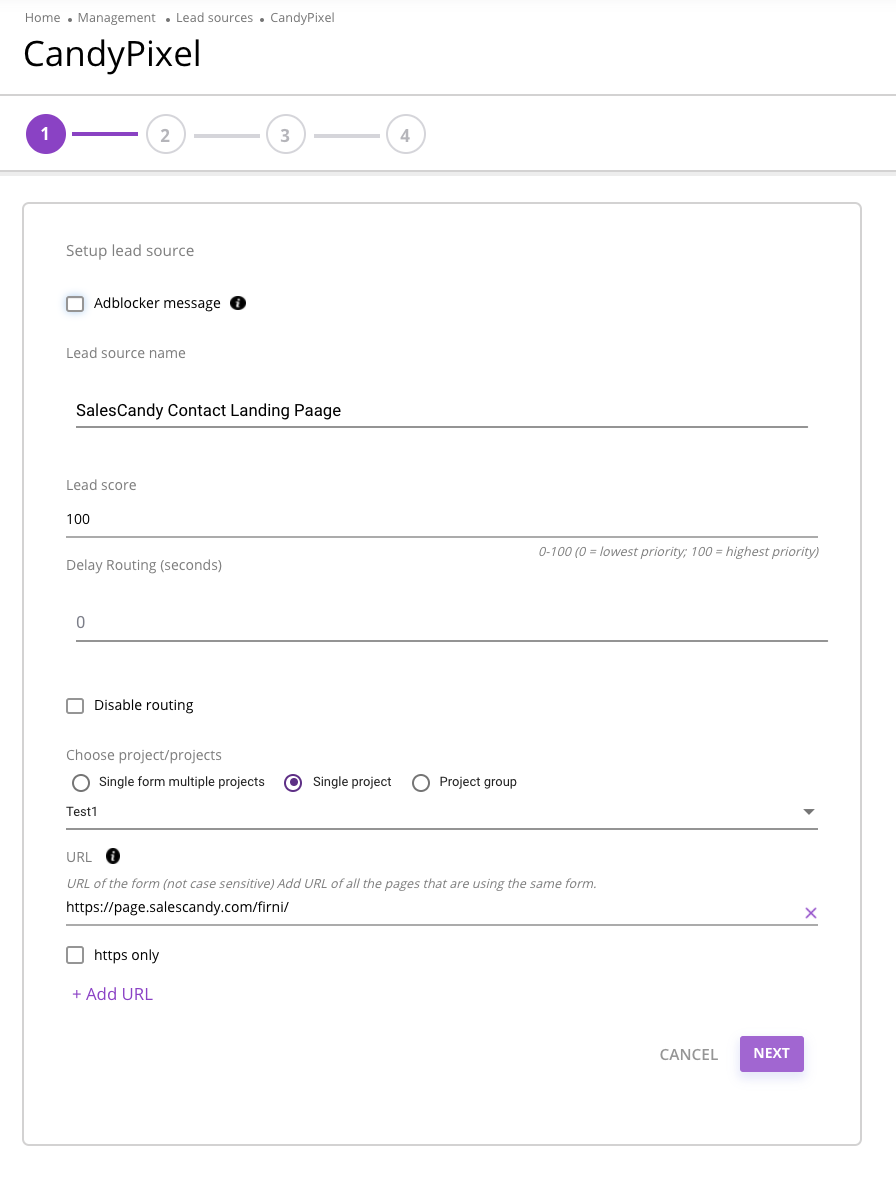The image shows a detailed screenshot of a form interface for inputting information. At the top, there are navigation headers: "Home" and "Management," followed by "Lead Source: CandyPixel" and "BlackTexas: CandyPixel," with both "C" and "P" in "CandyPixel" capitalized. 

A section features four circles numbered 1, 2, 3, and 4. The first circle is purple with an accompanying purple line, while the remaining circles are white with gray borders.

Further down, a box labeled "Setup Lead Source" is visible, offering a checkbox for "Add Block or Message." The form contains multiple fields:
- **Lead Source Name**: currently filled with "Sales, Candy, Contact, Landing Page."
- **Lead Score**: set at 100.
- **Delay Routing (Seconds)**: ranges from 0 (lowest priority) to 100 (highest priority). The current value is 0.
- **Disable Routing**: followed by options to "Choose Projects." The available options are "Single Form Multiple Projects," "Single Project," and "Project Group," with the current selection being "Test 1."
- **URL**: field for the form's URL, described as not case-sensitive, where users can add URLs for all pages utilizing the same form. An example URL provided is "https://page.salescandy.com/f-i-r-n-i/."

Additionally, there is an option labeled "HTTPS only" at the bottom of the form.